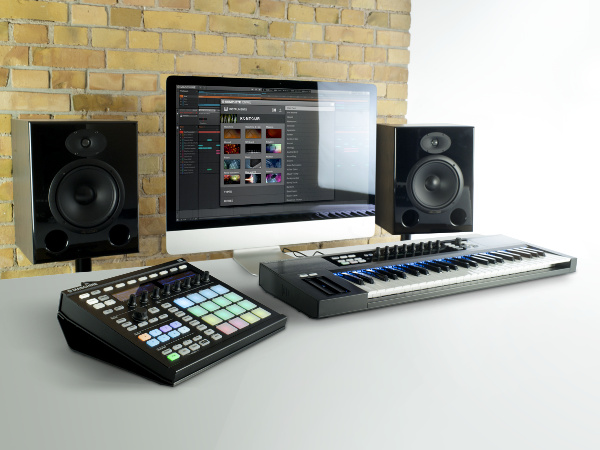The photograph captures a detailed indoor setup centered around a computer monitor positioned against a brick wall. Flanked by two large black speakers, the monitor is turned on, displaying an editing tool, though the screen image is slightly obscured by glare. In front of the monitor sits an electronic keyboard, distinctively a musical instrument rather than a computer accessory, with a black wire trailing off the desk, indicating it is plugged in.

To the left of the keyboard, there is an elaborate sound mixing system adorned with numerous colored buttons in shades of green, blue, and yellow, along with several dials and switches. The desk supporting these devices appears to be a white, flat surface. The area immediately to the far right of the monitor is marked by a patch of white void next to the brick wall, which stands out as though part of the photo is missing or cut out.

The photograph is well-lit, capturing the beige tones of the brick wall and a variety of colors from the equipment, including hints of blue, light blue, light green, light pink, light yellow, black, white, off-white, tan, maroon, teal, and purple. This vibrant and meticulously arranged do-it-yourself sound mixing station reflects a personal, creatively structured workspace.